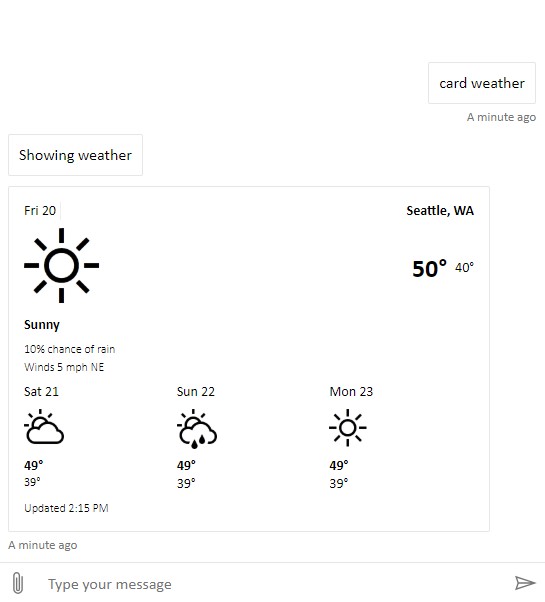The image displays a digital weather application interface on a white background with black icons and text. In the upper right-hand corner, there's a "Card Weather" label and a timestamp indicating it was updated "a minute ago." Directly below this, the text "Showing Weather" appears, followed by the date "Friday the 20th," beneath which an icon of a sun signifies bright, sunny weather.

On the left side of the screen, it specifies the location as "Seattle, Washington," with current temperatures listed as "50°F" and "40°F" in smaller text. Beneath the sun icon, it indicates a "10% chance of rain" accompanied by "winds at 5 miles per hour northeast."

Further down, three weather forecast icons for the upcoming days are displayed in a horizontal row. For Saturday the 21st, the icon shows partial sun with clouds, with temperatures of "49°F" and "39°F" below it. For Sunday the 22nd, the icon displays a sun partially hidden by clouds and raindrops, indicating light precipitation, with temperatures also at "49°F" and "39°F." Finally, for Monday the 23rd, the icon reverts to a sunny symbol with temperatures of "49°F" and "39°F."

At the bottom of the section, it mentions the last update time as "2:15 PM," with a small text note "a minute ago." At the very bottom of the screen, there's a small input box labeled "Type your message," flanked by a paperclip icon for attachments on one side and a navigation arrow on the far right to proceed to the next screen.